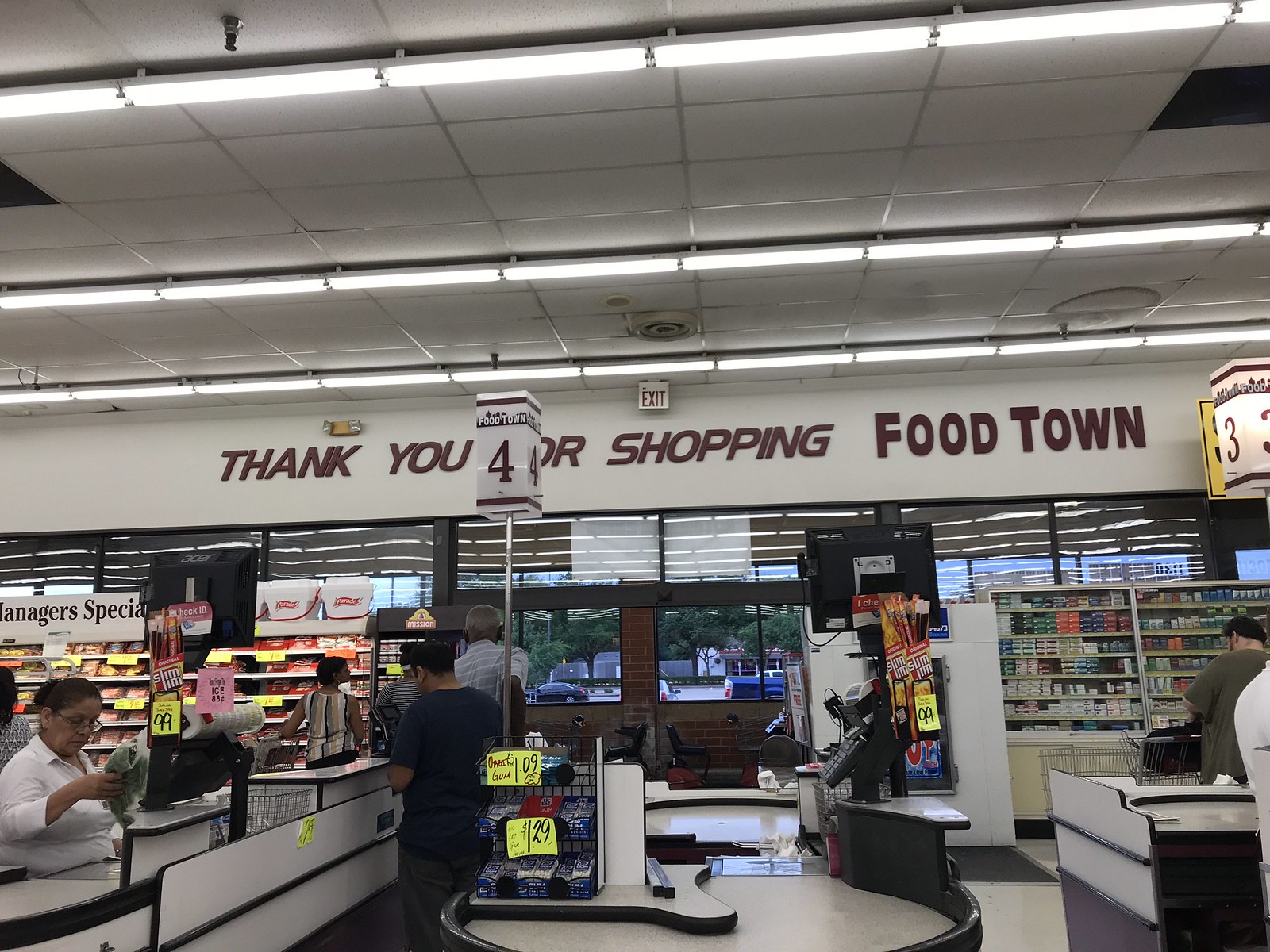This detailed photograph captures the bustling environment of a Foodtown grocery store's interior. The image, taken from the middle of the store, looks toward the main exit doors, beyond which a glimpse of the parking lot is visible through large windows. Dominating the upper portion of the image, a dark burgundy sign reads, "Thank you for shopping Foodtown," with some letters partially obscured by structures in the store. The ceiling features traditional white square tiles arranged in segments by gray lines, illuminated by three parallel strips of iridescent lights.

On the left side of the frame, several checkout counters are visible, staffed by cashiers and baggers assisting customers. One counter is clearly marked as cashier number three. Further back on this side, a sign announces a "Manager's Special," with products likely ranging from deli items to sandwiches or pastries displayed beneath it. In the center, aisle number four can be seen prominently. 

To the right, a large glass-fronted cabinet displays a variety of cigarettes securely locked up. Nearby, a shopper peruses a box of Slim Jim's priced at 99 cents. The bustling activity of the store is further highlighted by the presence of a ride-on shopping cart. Adjacent to the checkouts, CCTV monitors are placed to oversee the area. Overall, this scene epitomizes a typical day at Foodtown, illustrating the busy checkout counters, promotional signage, and security measures within the store.